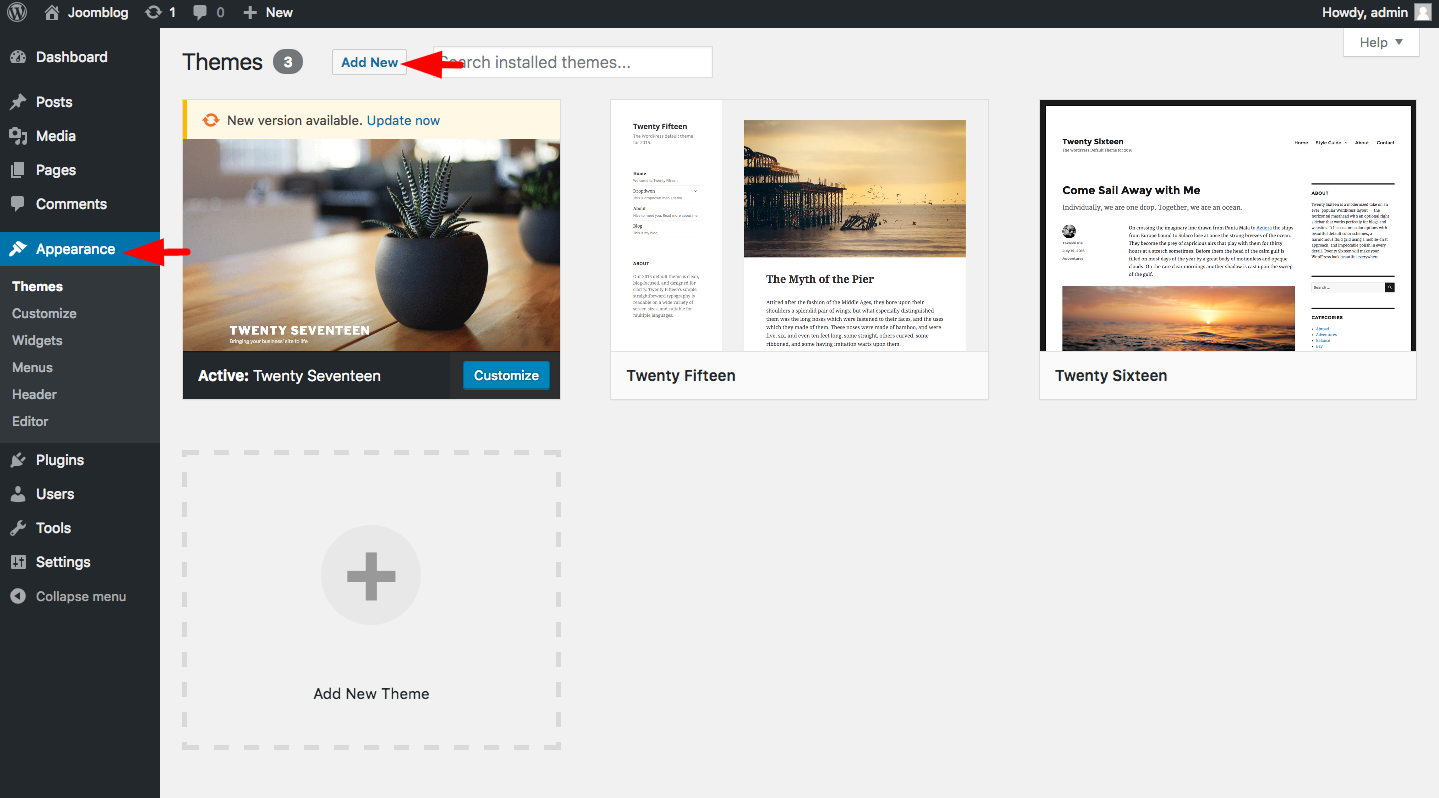This is a detailed screenshot of a blogging website identified as "Juneblog." At the top left corner, the site name "Juneblog" is prominently displayed. Directly beneath the site name, a navigation menu includes several options: Dashboard, Posts, Media, Pages, Comments, and Appearance, with "Appearance" highlighted. Within the highlighted Appearance section, additional sub-options are visible: Themes, Customize, Widgets, Menus, Header, and Editor, with "Themes" standing out in bright white text, indicating selection.

Below these options, further menu items are available: Plugins, Users, Tools, Settings, and Collapse Menu (in a darker gray color). 

The main section of the screen corresponds to the "Themes" option. Displayed are three currently available themes, each year-themed: "2017," "2015," and "2016." The active theme, denoted by a small black banner with the label "Active," is the "2017" theme, featuring an image of a black plant pot with a small plant growing from it. Options to add or install new themes are also present within this section, suggesting functionality for further customization.